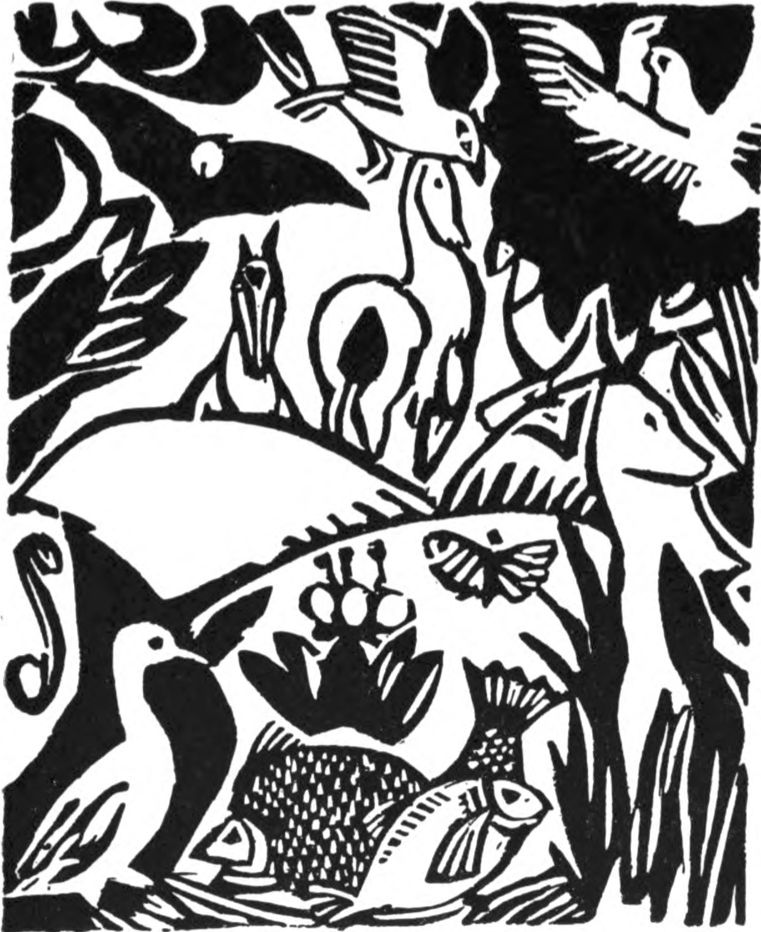This black and white art print, titled "Apollinaire Le Chantier Pourissant," is an intricate and imaginative depiction of a nature scene that feels almost like a fantasy jungle. The background is stark white, accentuating the heavy black lines that form a variety of animals and elements of the landscape. In the upper right corner, the sky is shaded black, creating a dramatic backdrop for two birds with their wings spread, facing each other. Below them, you can see other birds and bats with their wings open against the night-like sky. 

To the left, dark leaves encroach into the scene, beneath which a bat, silhouetted against what appears to be a moon, glides. The lower left corner reveals a snake, adding a hint of mystery to the composition. As you move your gaze across the image, you notice a duck, several fish both at the top and the bottom, and butterflies scattered throughout. The central and lower right sections feature deer peeking through the grass and horses in varying orientations—one with its rear facing us, displaying its flowing tail, and another facing forward.

The entire piece is rendered in an impressionistic, almost doodle-like style, giving it a whimsical yet sophisticated feel. The clever use of both heavy black lines and negative space creates a dynamic and engaging visual experience, making each animal and detail stand out individually while still blending into the harmonious whole of the artwork.